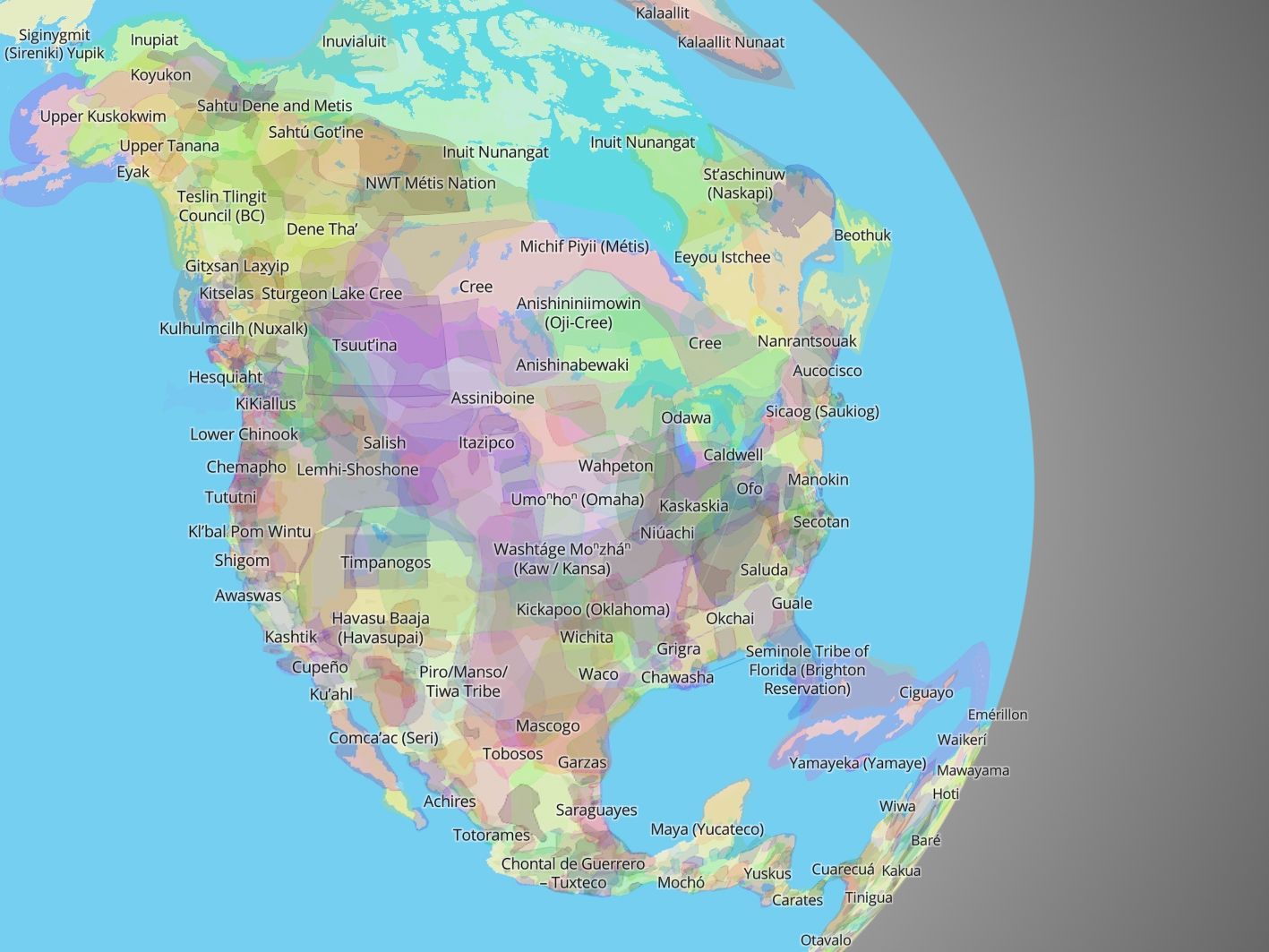This image showcases a highly contemporary and stylized section of a globe, focusing predominantly on North America and partially on South America and Antarctica. The map diverges from traditional representations by using a range of intertwining pastel colors to distinguish different areas. Unlike standard maps, the names on this globe do not correspond to conventional state or city names; instead, it features non-English, perhaps fictional, labels possibly indicating varied regions or tribes. Notably, familiar American names like Waco and Wichita appear amidst these unfamiliar ones. These labels are depicted in black text with a white outline. The entire illustration sits on a round, turquoise-colored globe, although the full globe isn't visible, and the image captures only the hemisphere containing the Americas.